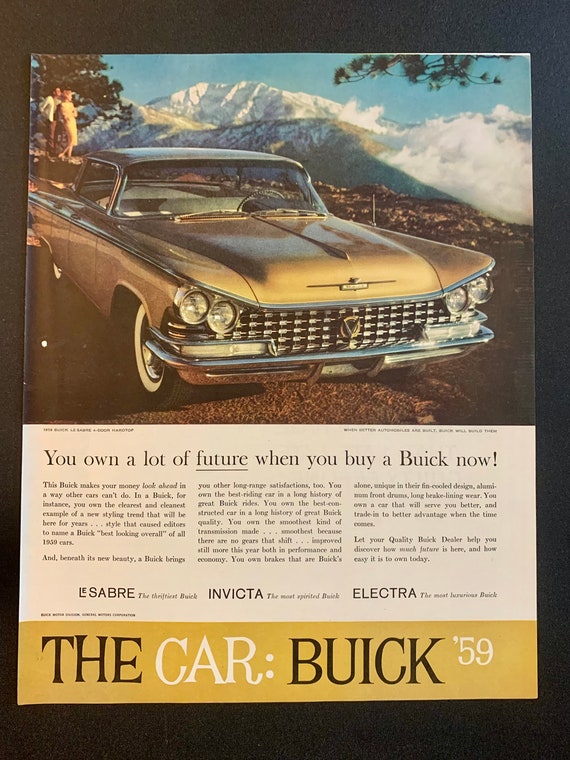This image is a vintage magazine advertisement for a 1959 Buick, featuring a gold-colored Buick prominently in the foreground with a gleaming silver grille. Behind the car, a couple stands on a rocky edge, gazing over a picturesque mountain range with scattered trees and snowy peaks. The headline below the photograph declares, "You own a lot of future when you buy a Buick now," emphasizing the forward-thinking design and value of the car. The advertisement also highlights the car’s advanced features and quality, noting its standout styling that won it accolades as the best-looking car of 1959. In addition to its aesthetic appeal, the ad details the superior construction, smooth transmission with no gear shifts, and unique braking system featuring aluminum front drums and extended brake lining wear. At the bottom of the page, a strip reads, "The car: Buick ’59," encapsulating the essence of this classic automotive promotion.